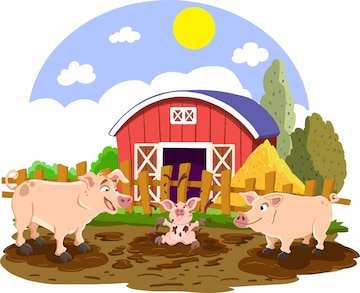The image showcases a vibrant cartoon artwork featuring a charming farm scene where a family of three pigs is playing in the mud. On the left side, a tall, pink male pig is looking downward with his mouth open. To the right, a shorter pink female pig with notably larger lips gazes towards the center. Between them, a baby pig, also pink, is joyfully sitting in an oval-shaped pool of mud, grinning widely as if experiencing the mud for the first time. Behind them, there's a round wooden fence that encloses the area, with a red barn that has a distinct dark blue, curved roof resembling an upside-down 'C'. Adjacent to the barn, on the right side behind the fence, there's a pyramid-shaped pile of hay. The backdrop features two green trees flanking the red barn and a semicircular sky with a bright yellow sun in the upper right corner, complemented by several puffy white clouds. The setting captures a delightful moment of family bonding amidst a picturesque farm landscape.